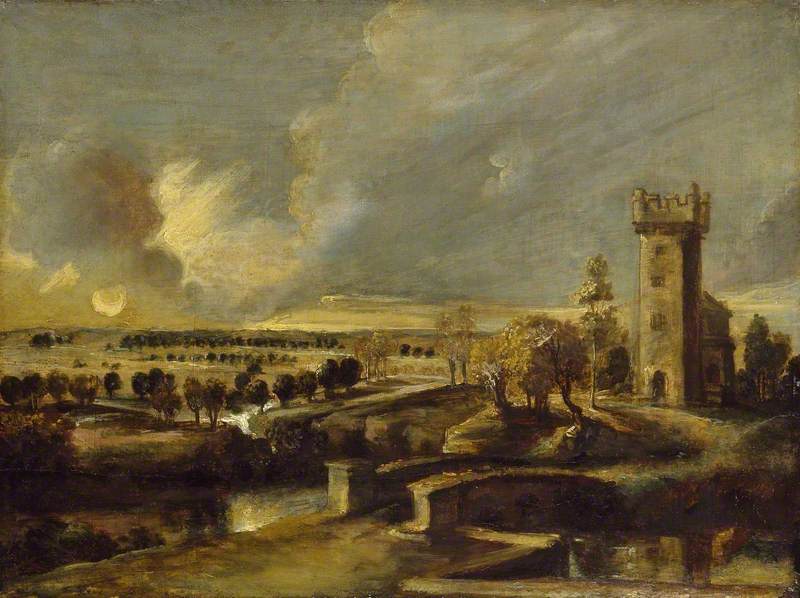This is a detailed painting rendered in dark tones of brown, gray, and beige, accentuated with white highlights and black contours. The scene captures a picturesque countryside with a prominent structure, possibly a church or castle, on the right side. This structure features a tall, square tower adorned with battlements, a large arched doorway, and three front-facing windows. Nestled behind it is a two-story stone building.

To the left, a stone arched bridge spans a tranquil river, leading to a pathway that winds through the bucolic landscape. The pathway meanders towards the tower and continues into the distance, where neat rows of green trees paint the rolling yellow hills.

The expansive sky, occupying the upper half of the rectangular canvas, is a moody gray filled with large, dark gray and white clouds, with occasional streaks of brown and hints of mustard yellow. The sky and the landscape are depicted with visible, somewhat unfinished brushstrokes, adding a dynamic, textured feel to the piece. The entire painting, measuring about 6 inches wide by 4 inches tall, reflects an old style, capturing the serene yet evocative essence of the countryside.